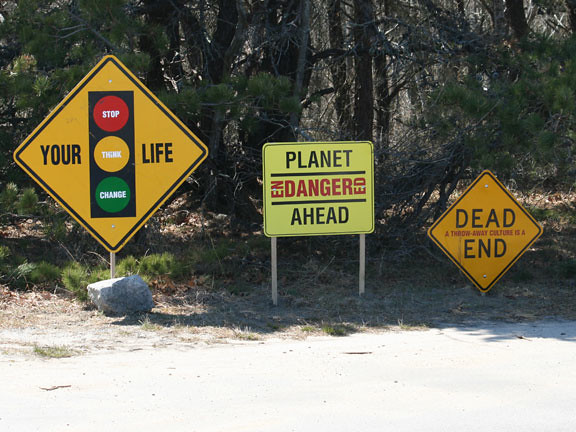This image showcases a series of traffic and warning signs displayed along a pavement path, with the sun casting shadows from surrounding large trees, including some evergreens with prominent trunks. 

The first sign on the left is diamond-shaped with a yellow background and black border. It features a traffic light symbol indicating the sequence of lights: a red circle labeled "STOP," a yellow circle labeled "CAUTION," and a green circle labeled "GO." This sign is mounted on a stake planted in the ground, with a large gray rock positioned directly in front of it.

To the right of this traffic light sign is a square sign with a warning message that reads, "Planet Danger Ahead." The "EN" in "PLANET" and "ED" in "DANGER" are angled differently from the rest of the text, giving a unique appearance to the sign.

The third sign in the sequence is another diamond-shaped sign with red lettering that reads "DEAD END." The sign also has some additional text in the middle, though it is too blurred to decipher. This set of signs is grounded near a paved area under a clear, sunny sky.